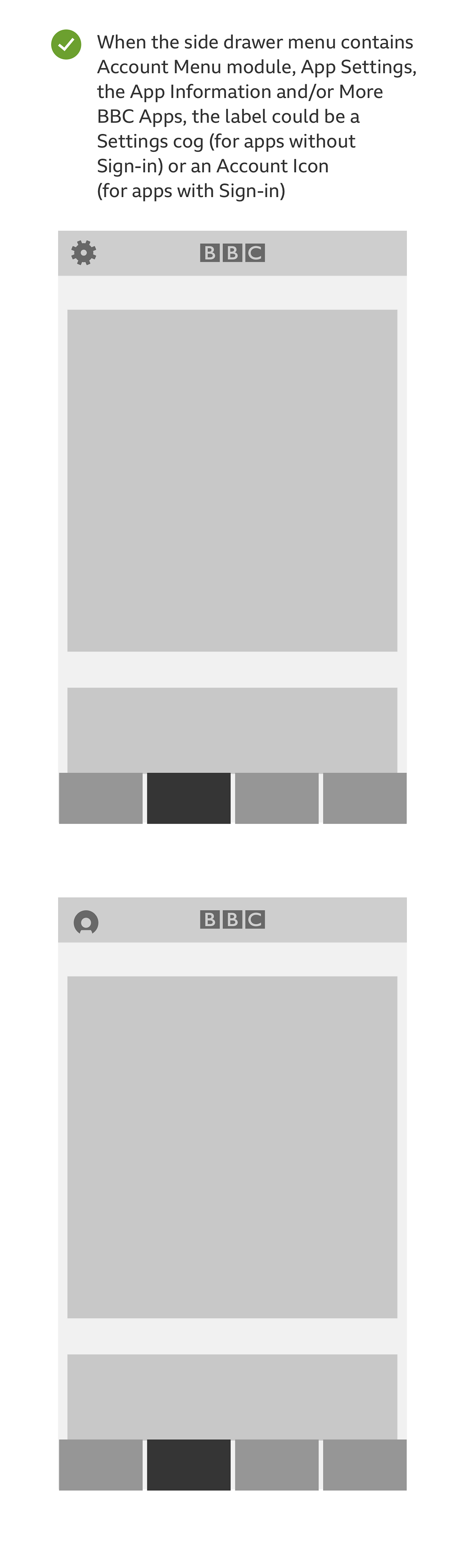The image features two grayed-out mobile app screens, stacked vertically, portraying different interface designs based on user sign-in status. 

Above these screens, a green checkmark precedes explanatory text. The message is as follows: "When the side drawer menu contains account menu module, app settings, app information, and/or additional BBC apps, the label could either be a settings cog for apps without sign-in or an account icon for apps with sign-in."

Below this text, the first grayed-out screenshot is displayed. In the top left corner, a settings icon is visible beside the BBC logo. This screen is populated with various gray boxes of different sizes and shades, indicative of placeholder content.

The second screenshot, positioned directly beneath the first, mirrors its design except for a notable difference: the top left corner features an account login icon instead of a settings icon.

Both screenshots have four rectangles spanning the bottom width of the screen. In each image, the second rectangle from the left is darker than the other three, possibly highlighting the active tab or section.